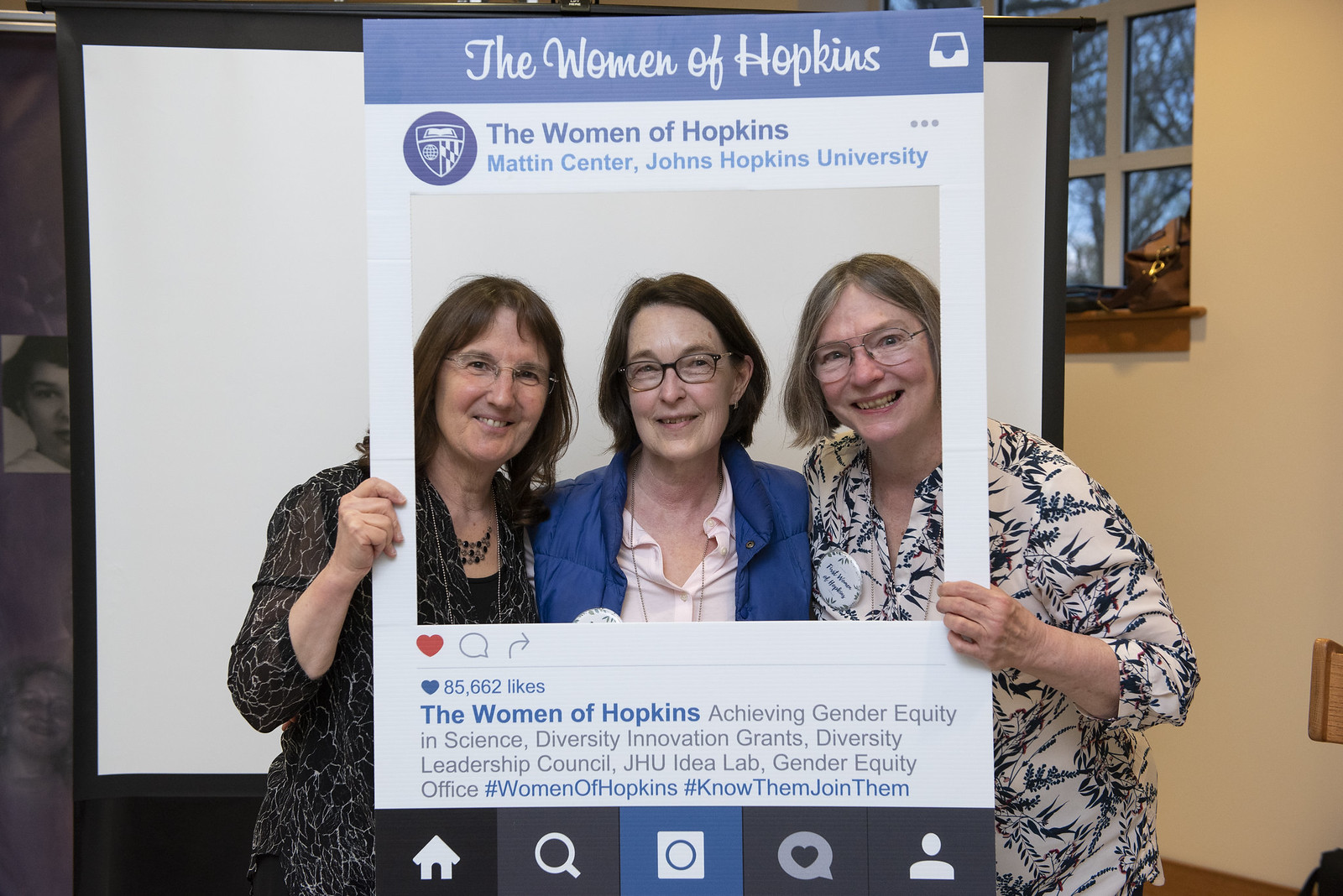In this vibrant photograph, three middle-aged women are participating in a charity event, captured in a playful and creative manner. They are posing with a large printout designed to look like an Instagram post, adding a fun and modern twist to the traditional group photo. The faux Instagram frame at the top reads "The Women of Hopkins" with a location tag indicating the Matten Center at Johns Hopkins University. The post has garnered an impressive 85,662 likes. The accompanying text highlights important initiatives such as "Achieving Gender Equity in Science," "Diversity Innovation Grants," "Diversity Leadership Council," "JHU Idea Lab," and the "Gender Equity Office." The hashtags #WomenOfHopkins and #KnowThemJoinThem further emphasize the post's focus on promoting gender equity and community engagement.

The women in the photo, each exuding a sense of pride and camaraderie, are dressed in casual yet stylish attire. On the left, a woman with shoulder-length brunette hair wears a simple black top. The woman in the middle, who appears to be the most understated yet equally joyful, sports shoulder-length hair, glasses, and a cozy blue puffy jacket over a button-down shirt. On the far right, the most exuberantly smiling woman is adorned in a tan and black floral-patterned blouse. The two women on the ends hold up the striking Instagram printout, framing their faces and adding an interactive layer to the image.

This descriptive caption not only paints a vivid picture of the scene but also underscores the meaningful cause they are championing: promoting gender equity at Johns Hopkins University.